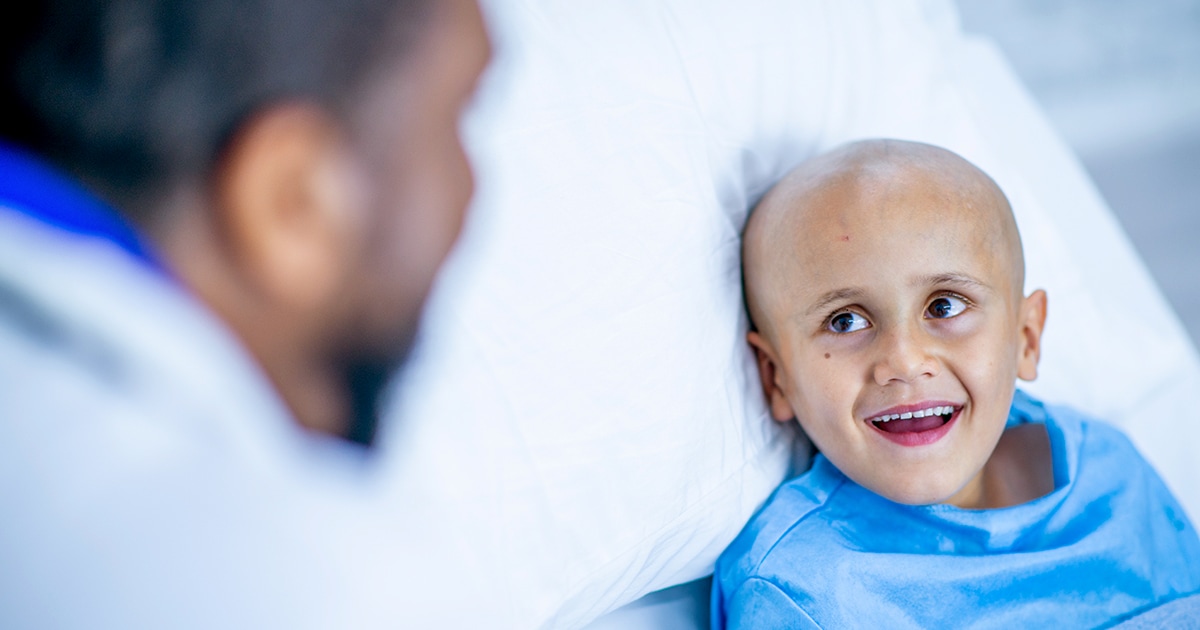The photograph captures a tender moment in a hospital room, featuring a young child with a bald head, likely undergoing cancer treatment, lying in a hospital bed. The child, dressed in a blue hospital gown, rests their head on a white pillow and smiles warmly, revealing small teeth, at a bearded doctor standing nearby. The doctor, seen in profile with graying black hair and a brown beard, is dressed in a white lab coat with a vibrant electric blue shirt peeking out underneath. He appears to be engaging with the child in a way that brings comfort and joy, creating a heartwarming and endearing scene that underscores his caring bedside manner.